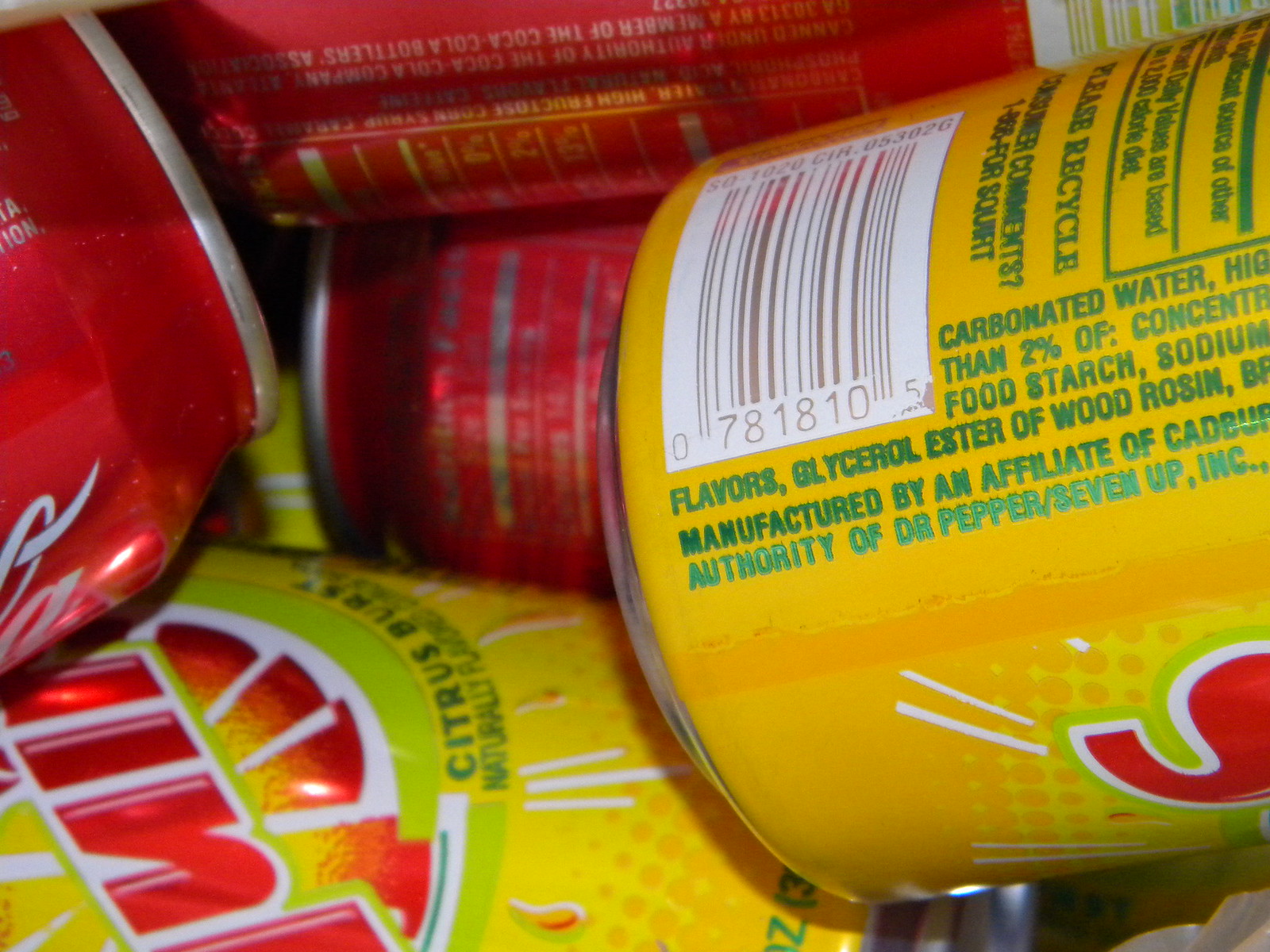This rectangular photograph, dominated by artificial light, captures a cluster of aluminum soda cans with their long side extending from left to right. Prominently featured in the foreground are two vivid yellow cans of Sun Citrus Burst Soda, with "Sun" written in red text. The nutritional information on these yellow cans is highlighted in green text, stating ingredients such as carbonated water, fruit starch, sodium, flavors, glycerol, ester of wood rosin, and a UPC code (07818105) in dark brown or gray text on a white background. Interspersed among these yellow cans are several red cans, identifiable as Coca-Cola, with part of the name visible, particularly the "L-A" at the edge of one can. All cans share the characteristic silver rims along their round edges. The entire arrangement suggests an indoor scene, further accentuated by the glow of artificial lighting.